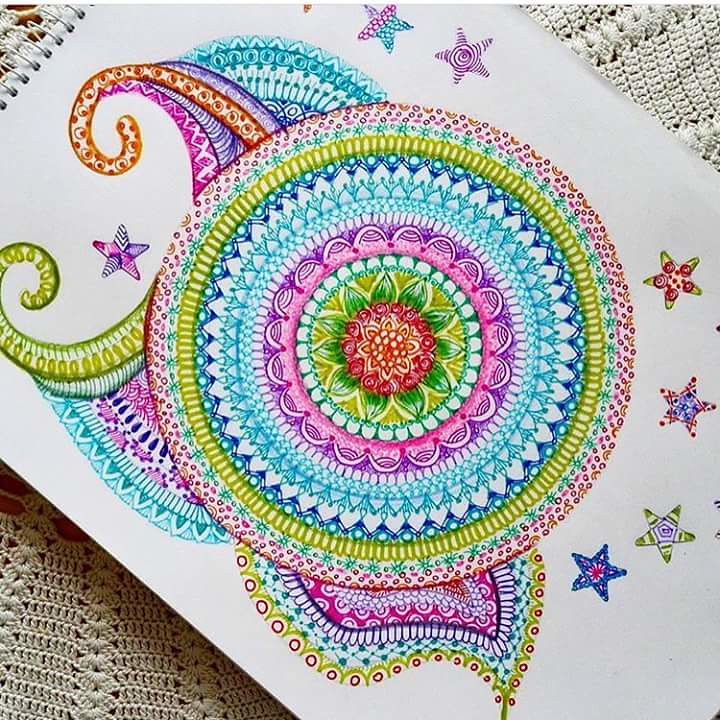A detailed and vibrant mandala drawing is prominently displayed on a diagonally positioned 8 1⁄2 by 11-inch sketchbook with white paper. The mandala is an intricate and colorful design that begins at the center with a pink and red flower accented by orange hues. Surrounding the flower are green leaves and green stripes, leading to a scalloped aqua border. This is followed by a ring of purple scallops and then teal mandala designs accentuated by a darker blue ring. The design transitions back to aqua, then features more green elements, aqua sun shapes, pink dots, and purple small circles, with additional orange or red accents. The mandala is complex, with various elements including stars and paisley designs that have leaf-like shapes and curly cues extending outward in a neon color palette dominated by pinks, purples, oranges, greens, and blues.

In the background, there is a white, machine-knit lace tablecloth placed on a wooden surface, which is partially visible through the lacework. The tablecloth adds a delicate, textured element to the scene, contrasting with the bold mandala design. The overall composition creates a rich, detailed, and colorful visual experience.